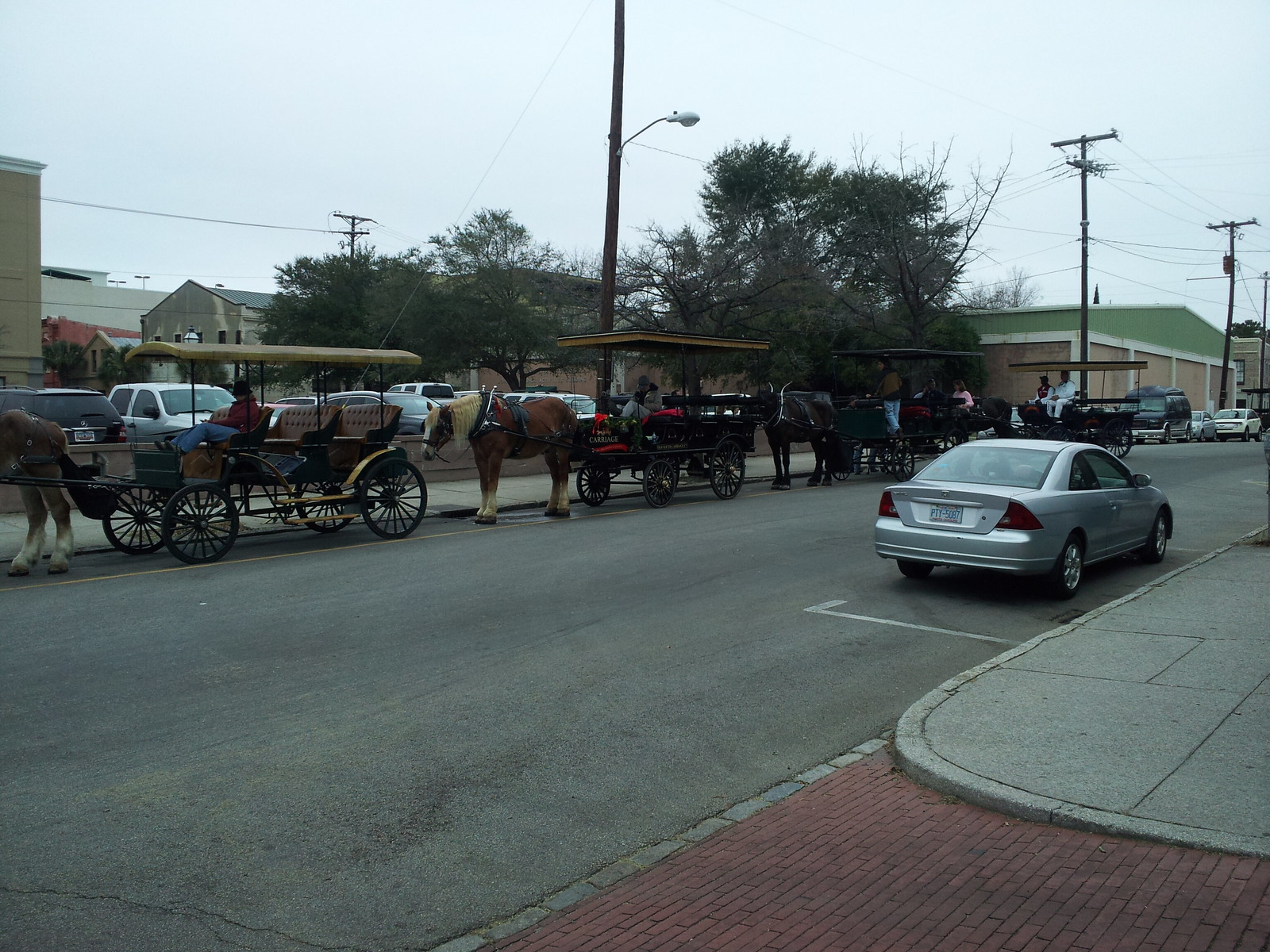The photograph captures a nostalgic yet modern outdoor scene depicting a procession of four horse-drawn buggies on an asphalt road. The gray sky above is overcast, casting a muted light over the scene. Each of the buggies, complete with a four-wheeled carriage, has a distinct horse in harness—most visibly, a brown horse with a blonde mane and tan legs. Alongside the buggies, people are either sitting inside or standing next to them, adding a sense of community to the image. On the right-hand side of the road, a silver sedan is parked, its rear and side clearly visible with a white outline marking its parking space. Below the car, there's a gray sidewalk, and adjacent to it, a red brick walkway adds a splash of color. In the background, a row of small buildings is seen, most notably a brown structure with a green roof, surrounded by trees with dark green leaves. Light poles, power lines, and utility poles run parallel to the sidewalk and the road, blending the old-fashioned scene of buggies with modern urban elements.